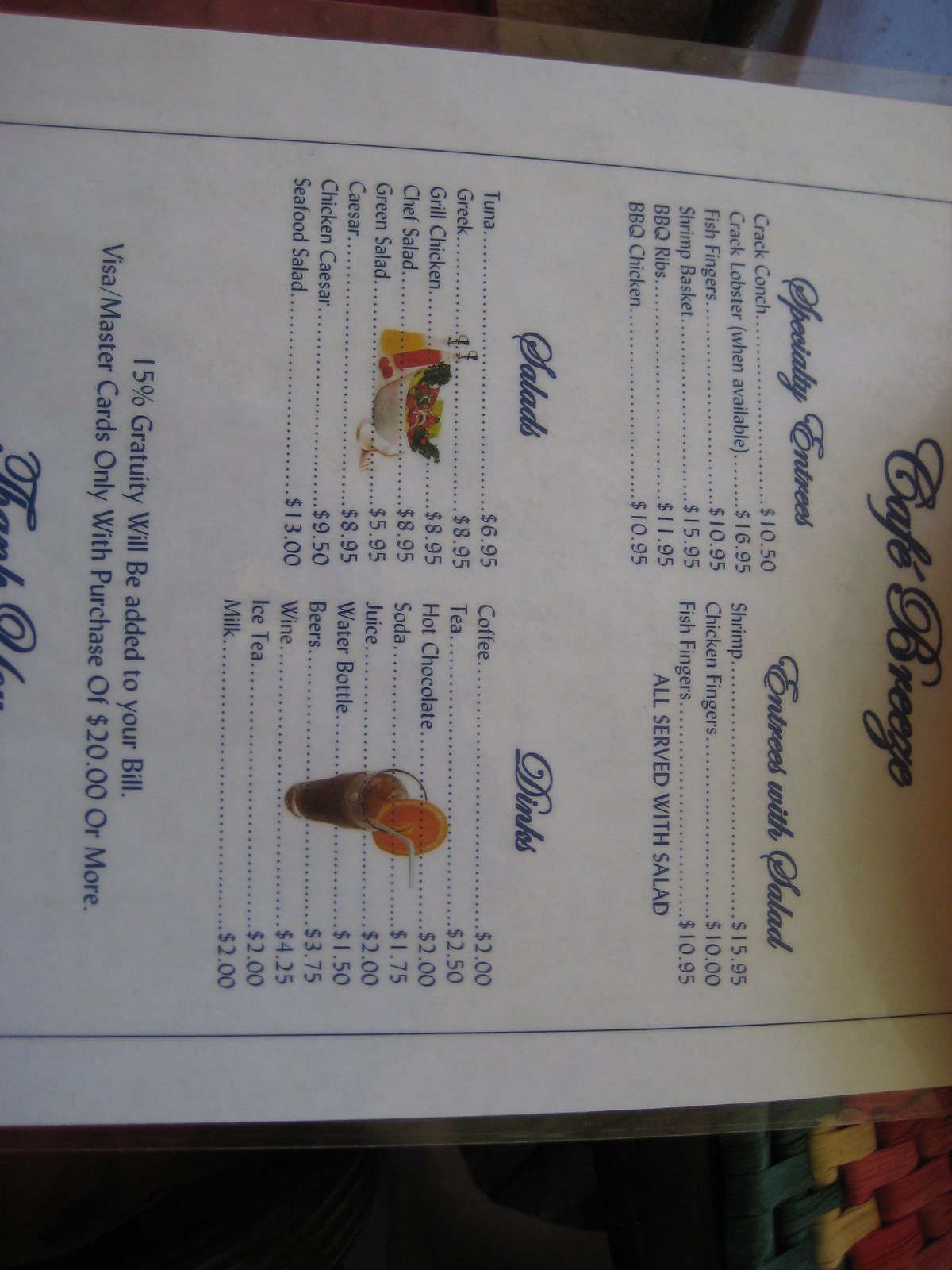This image captures a restaurant menu from Cafe Breeze, oriented sideways with the top of the menu on the right and the bottom on the left. The menu prominently displays categories including Specialty Entrees, Entrees with Salad, Salads, and Drinks. The featured images in the center of the menu include a vibrant salad accompanied by various dressings and a refreshing drink garnished with an orange slice and a straw. 

In the Drinks section, options such as coffee, tea, hot chocolate, soda, juice, bottled water, various beers, wine, iced tea, and milk are listed, each with their respective prices. The Salads section includes a diverse range like tuna, Greek, grilled chicken, chef salad, green salad, Caesar, chicken Caesar, and seafood salad, with prices clearly listed beside each option. This detailed menu from Cafe Breeze offers a variety of appetizing choices for its patrons.